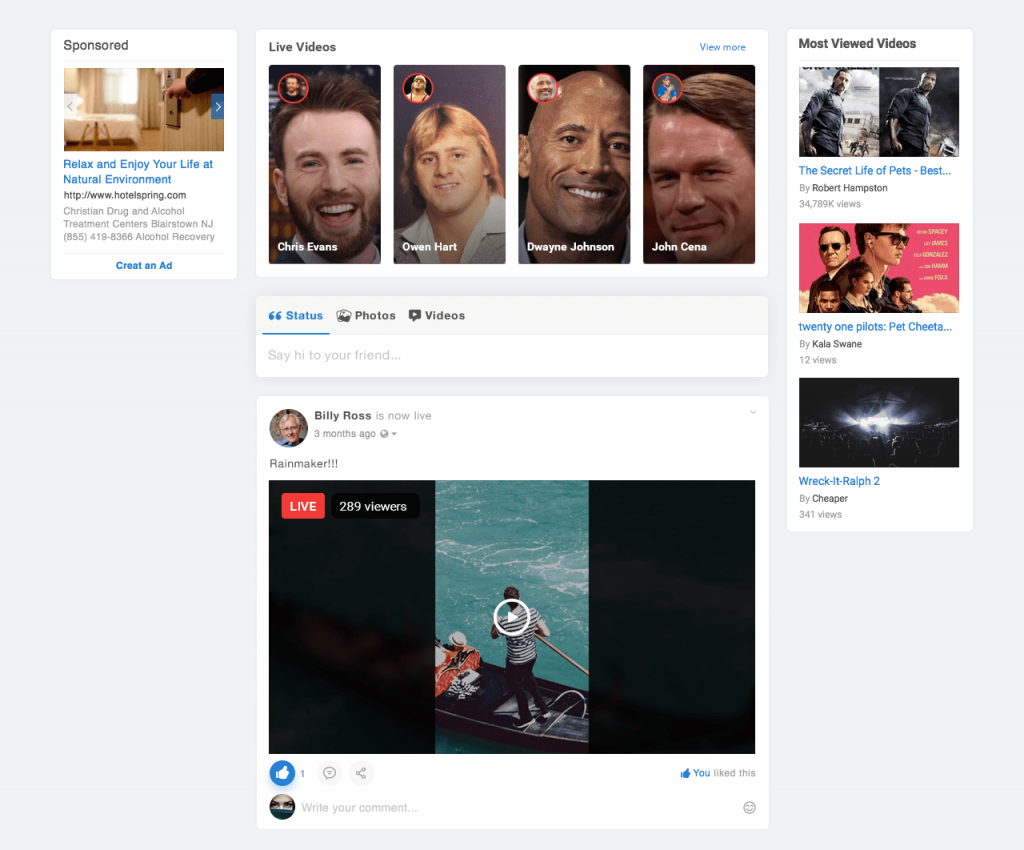Screenshot of a Facebook feed showcasing various live events and posts:

- **Top Section**: The toolbar at the top-center includes settings and options for live videos.
- **Live Videos Section**: 
  - The center of the image features a Facebook feed with four live video squares, each showing a famous personality.
  - **Top Left Square**: An image of Chris Evans.
  - **Top Right Square**: An image of Owen Hart.
  - **Bottom Left Square**: An image of Dwayne Johnson.
  - **Bottom Right Square**: An image of John Cena.
  
- **Post Section**: 
  - Below the live video squares, there is a post from Billy Ross with the caption "Rainmaker".
  - Accompanying the post is a video depicting a man standing in a gondola, ferrying passengers through the canals of Italy.

- **Sponsored Ad**: 
  - On the upper left side of the page, there is a sponsored ad featuring a person opening a hotel room door with the tagline "Relax and enjoy your life in a natural environment."

- **Most Viewed Videos**: 
  - On the upper right side of the page, there is a list of the most viewed videos.
  - **Top Video**: "The Secret Life of Pets".
  - **Second Video**: "21 Pilots".
  - **Third Video**: "Wreck-It Ralph 2".

This detailed caption highlights the various elements present in the Facebook feed screenshot, providing a comprehensive description of each segment.